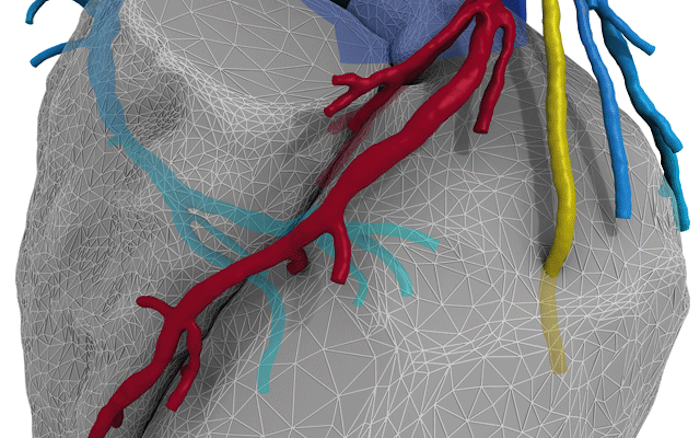The image showcases a detailed 3D model of a heart and its surrounding veins and arteries, created using a 3D modeling program. The heart is represented as a gray mass composed of numerous connected triangular polygons, which vary in size and density to illustrate different textures and levels of detail. Areas requiring more intricate detail feature smaller, closely packed triangles. The model also includes veins and arteries depicted in vibrant red, yellow, and blue hues. These vein and artery structures are partially integrated into and wrapped around the heart model, reinforcing its anatomical accuracy. The entire rendering highlights the complexity of the heart’s structure, with the use of color and polygon shapes enhancing the visual clarity and educational value of the model.